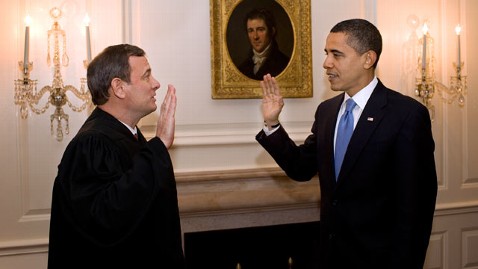This digital screenshot captures an interior view of the White House, offering a glimpse into the historical context and decorum of the setting. The room features an elegant wood-paneled white background, adorned with opulent, gold and silver-toned chandeliers mounted on the walls, each holding two candle-like electric light bulbs that enhance the grandeur of the scene.

Central to the image is an ornate gold picture frame housing a portrait of an unidentified, formally dressed white gentleman. Beneath the portrait, a cream-colored mantle frames a partially visible fireplace opening, adding a touch of classic refinement to the room.

On the left side of the image, a white man with predominantly dark, salt-and-pepper hair, dressed in a white robe, is seen raising his hand. Opposite him, on the right side of the frame, stands then-President Barack Obama, characterized by his short black hair and light skin tone. Dressed in a dark navy or black suit, paired with a white collared shirt and a striking light purple tie, he mirrors the other man's gesture by raising his own hand near the fireplace.

This moment captures the reenactment of President Obama's presidential oath-taking ceremony. The redo was necessitated due to an earlier error in the recitation of the oath, ensuring the legitimacy and correctness of his inauguration.